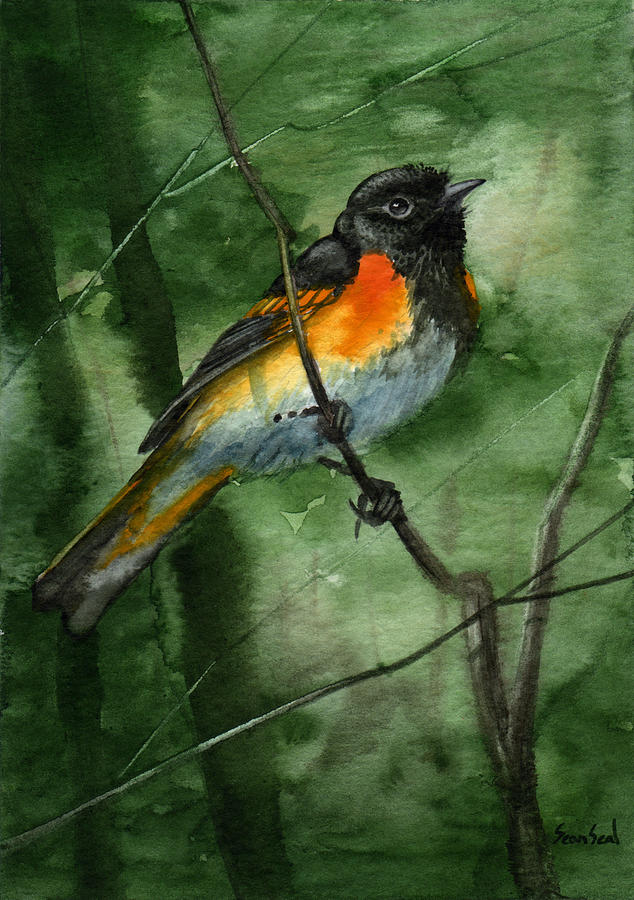This detailed watercolor painting showcases a bird perched on a branch against a predominantly green background. The bird, likely a cowbird, features a white breast, a black crown, and a black beak, with striking black feathering accented by orange and yellow spots on its sides and tail. Its long tail, which includes shades of orange, white, and black, complements its overall intricate coloring. The bird is depicted in a resting position with closed wings and a closed beak, oriented towards the right side of the image, adding a sense of tranquility to the scene. The background is lush and green with varying shades and shadowing, emphasizing the bird as the central focal point. The branch it perches on is brown and barren of leaves, enhancing the bird's vivid colors. The artist's signature, "Sean Seale," is noted in black at the bottom right of the painting, adding a personal touch to this realistic and detailed artwork.